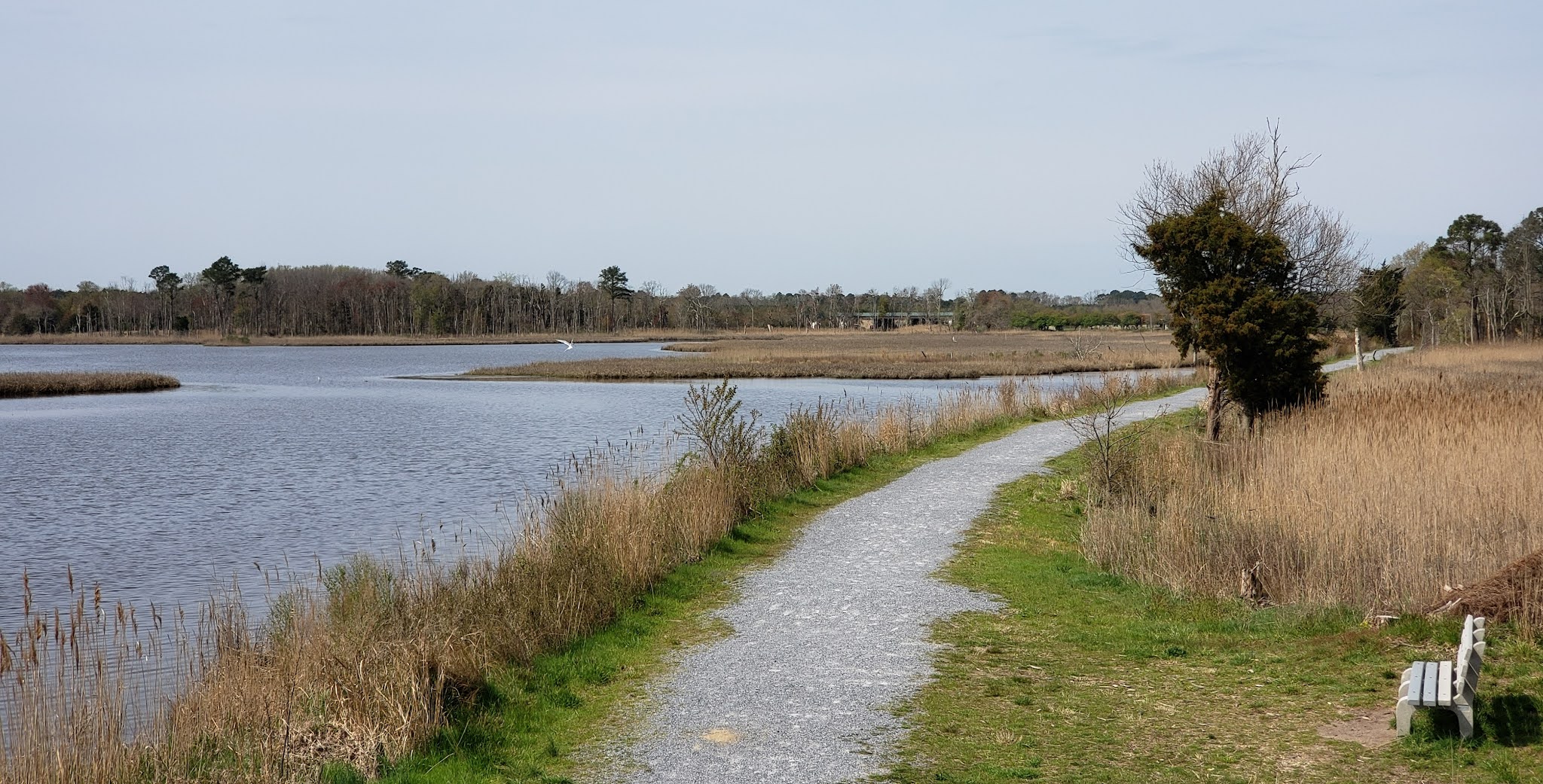The image captures a serene path made of gravel that winds alongside a picturesque lake. The left side of the image features the dark blue waters of the lake, bordered by various edge-of-the-water plants including cattails, brown foliage, and a small green plant. A green and brown grassy strip separates the path from the water. In the background, a distant shoreline is visible, dotted with a mix of tall trees—some bare and some evergreen—as well as a couple of small islands with vegetation.

On the right side of the path, a large field filled with tall brown stalks and patches of green grass extends into the distance. A gray bench, likely made of wood and painted white and gray, sits invitingly in front of this field. There is a single tree with green leaves standing alone in the middle of the field, adding a focal point to the landscape. The path curves up and to the right, flanked by more green grass with splotches of brown, leading towards a secluded cluster of evergreen and leafless trees. The sky above is a subdued cyan with a gray overcast, setting a tranquil, reflective mood.